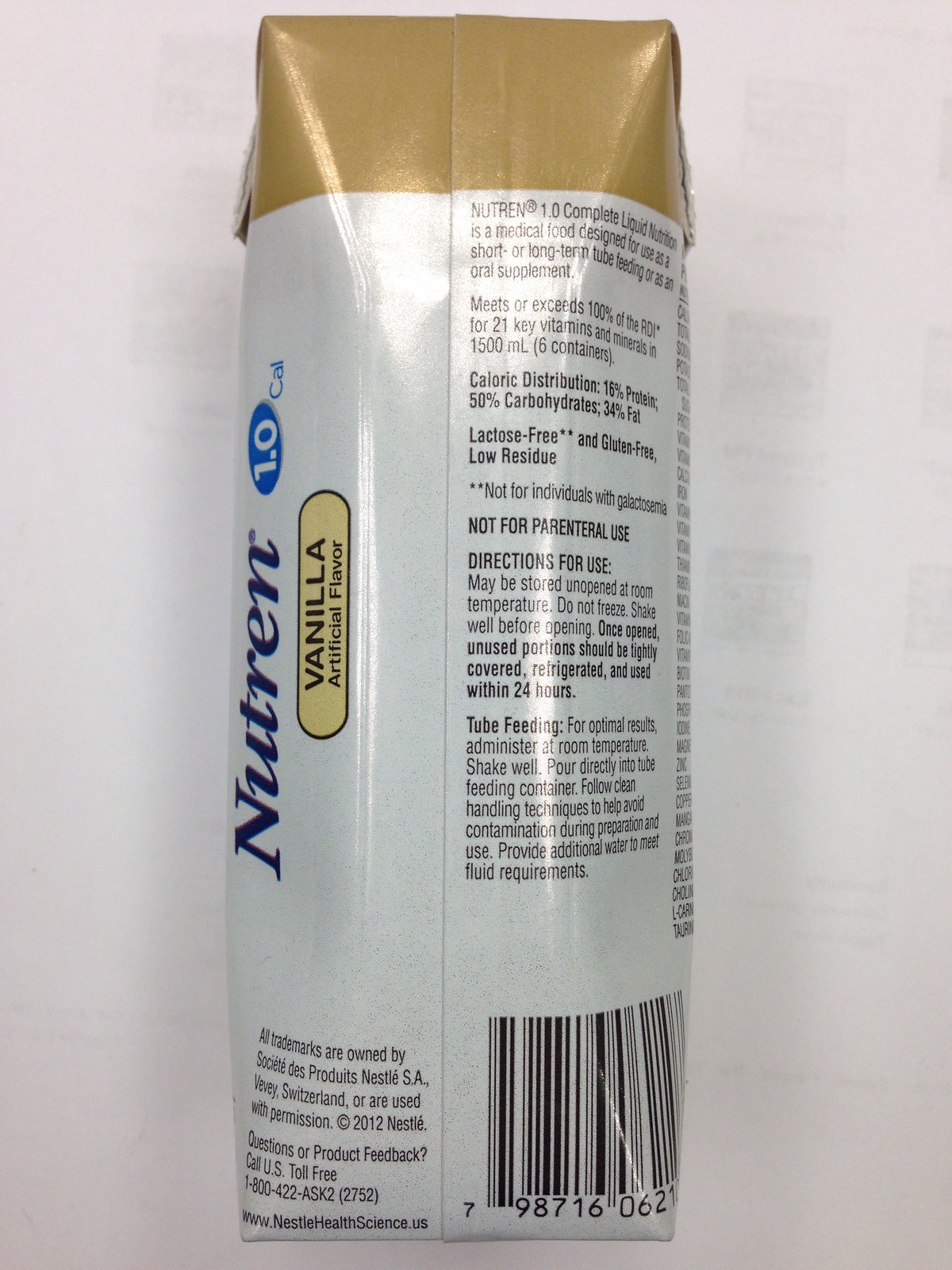The image displays the back of a Nutren 1.0 Complete Liquid packaging with black lettering on a white background. Central to the design is a capsule-shaped bar labeled "Vanilla Artificial Flavor" on a tan background. Adjacent to it, the text reads "1.0 CAL." The top of the package is gold, with "Nutren 1.0 Complete Liquid" clearly marked.

The product is described as a medical food designed for short or long-term tube feeding or oral supplementation. The text states that it meets or exceeds 100% of the recommended daily allowance for essential vitamins. The caloric breakdown is detailed as 16% protein, 50% carbohydrates, and 34% fat. Additionally, it is specified as lactose-free, gluten-free, and low-residue.

A caution note mentions, "Not for individuals with," followed by an unreadable word, and "Not for parenteral use." Below this, the text provides directions for use, specifically for tube feeding. A UPC code is positioned at the bottom, and to the left, there is contact information for customer inquiries.